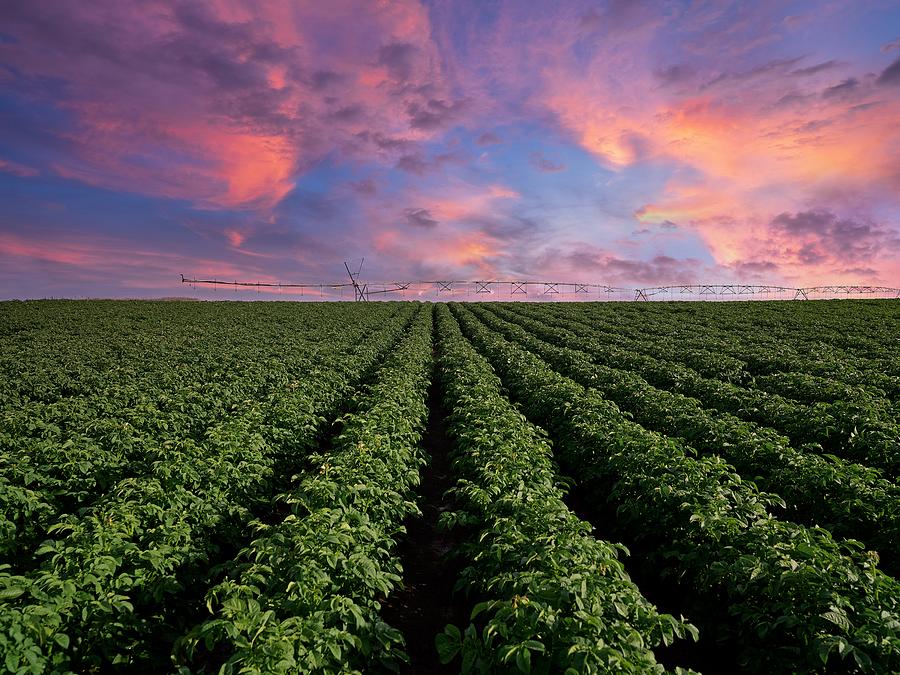The photo depicts an expansive crop field, characterized by rows of lush, green leafy plants that stretch symmetrically from the foreground to the distant horizon. The field is meticulously maintained, with its verdant vegetation closely hugging the earth in parallel lines. Towards the horizon, there appears to be a thin structure, possibly a bridge, trestle, or aqueduct, crossing the width of the field. Above this green expanse, the sky is a strikingly rich blue, accented with clouds in varying shades of pink, yellow, and orange, suggesting a breathtaking sunset. The interplay of colors in the sky contrasts vividly with the green below, adding a dramatic and serene quality to the panoramic outdoor scene.